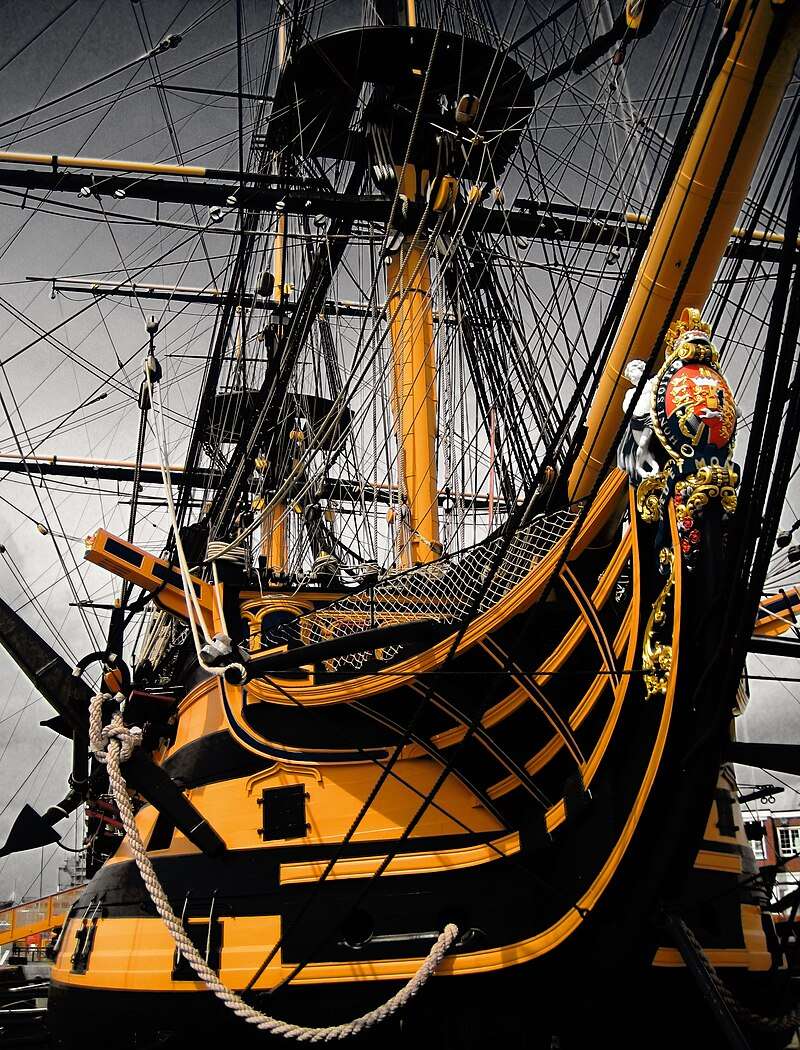The photograph captures a remarkably large, intricately designed ship, prominently featuring a curved bow adorned with an elaborate carved emblem. The ship, potentially a modern replica of an old schooner or a historically styled vessel, showcases a metallic gold and red color scheme with intricate details including what appears to be a coat of arms and a small statue, possibly of a baby or a small figure. The hull and structural components are primarily black and orange, with orange poles ascending through a chaotic web of criss-crossing cables and rigging that extend across the ship, contributing to a sense of organized complexity. The ship, docked in a harbor, is surrounded by a cloudy sky, adding a dramatic backdrop to its vivid and detailed appearance. The paint looks new, suggesting the ship may be a contemporary recreation designed to mimic the aesthetics and grandeur of historical maritime craftsmanship.